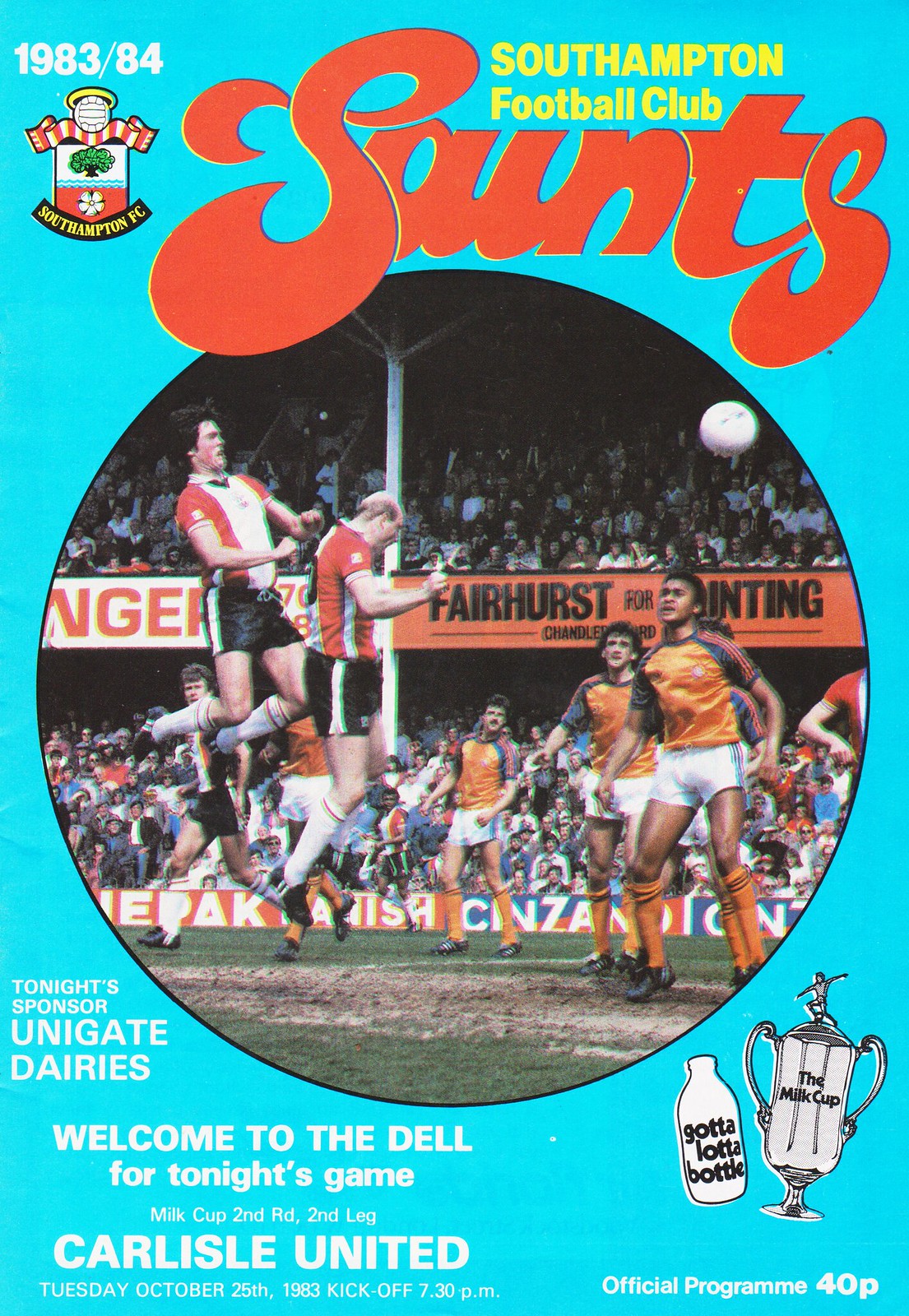The cover of this official program, set against a bright sky-blue background, prominently features "Southampton Football Club" in yellow font at the top right, with the bold red 70s-style "Saints" directly below. On the left side, the season "1983-84" and the Southampton FC crest are displayed. The central focus is a round black-framed photo capturing an intense soccer match between two teams—one in red with black shorts and the other in orange with black sleeves, white shorts, and orange socks. Several players are seen jumping, eyes fixed on the ball located at the top right of the image. The bottom left of the cover bears the white text: "Tonight's Sponsor, Unigate Dairies. Welcome to the Dell for Tonight's Game. Milk Cup 2nd Round, 2nd Leg, Carlisle United. Tuesday, October 25th, 1983, kickoff, 7.30pm." Additionally, there's a fun cartoon at the bottom right showing a milk cup and a milk bottle with "got a lot of bottle" written on it, beside the text "Official Program 40P."